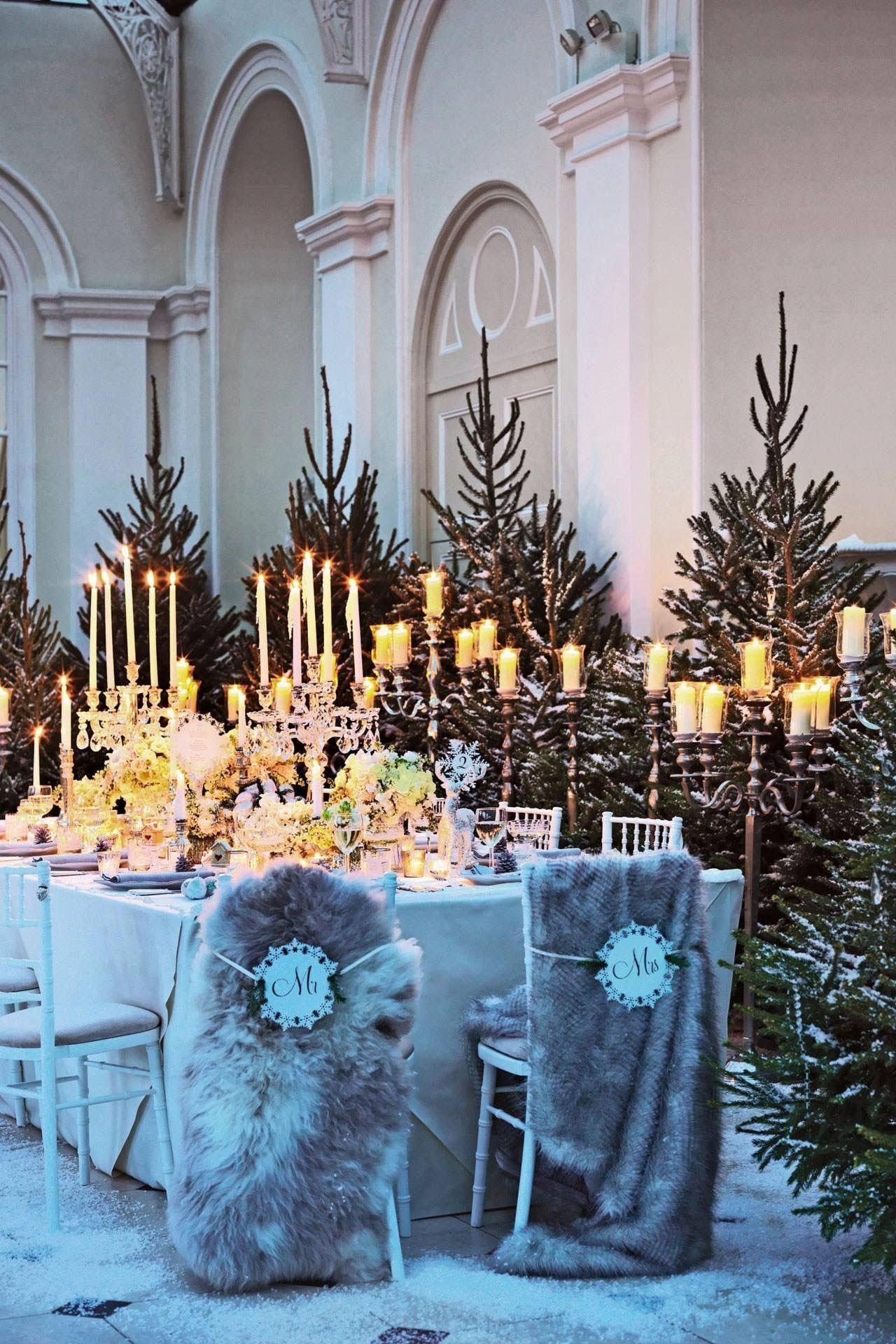This image captures an elegantly prepared wedding reception in an ornately decorated room with high ceilings, intricate crown moldings, and elaborate latticework where the walls meet the roof. The ambiance is strikingly winter-themed, featuring tall, snow-dusted pine trees reminiscent of a Christmas wonderland. The table is adorned with numerous candles, including tea lights and two large candelabras that are festooned with large crystals, casting a soft, enchanting glow over the scene. The table also showcases fine china and meticulously arranged place settings, amplifying the sense of luxury. White chairs with gray upholstered seats surround the table, while the head of the table features two special chairs adorned with faux fur stoles, marked with "Mr." and "Mrs." signs attached by elegant bands. The entire setup exudes a festive and romantic atmosphere, ready to welcome the bride, groom, and their guests.